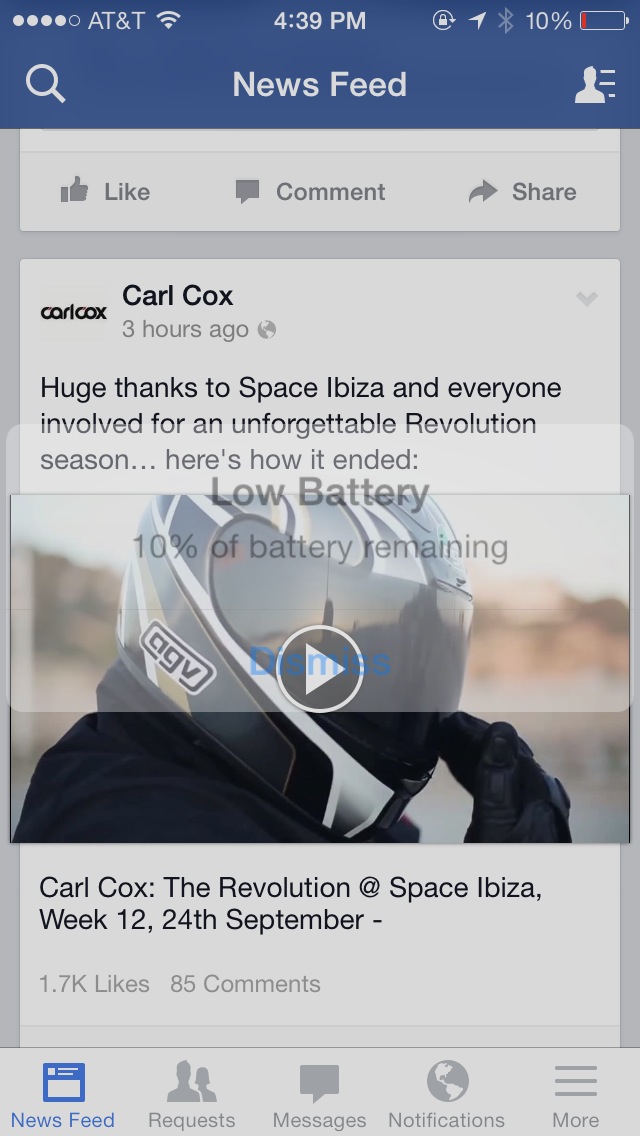The screenshot depicts a smartphone displaying a Facebook news feed at 4:39 p.m. on the AT&T network, with a Wi-Fi connection, 10% battery life remaining, and a low battery notification appearing faintly. The main visible post is from Carl Cox, posted three hours ago, thanking Space Ibiza and everyone involved for an unforgettable revolution season. It includes a video thumbnail showing a person in a motorcycle helmet raising a hand to their helmet. Below the thumbnail, the text reads: "Carl Cox, the revolution at Space Ibiza, week 12, 24 September." The post has garnered 1.7K likes and 85 comments.